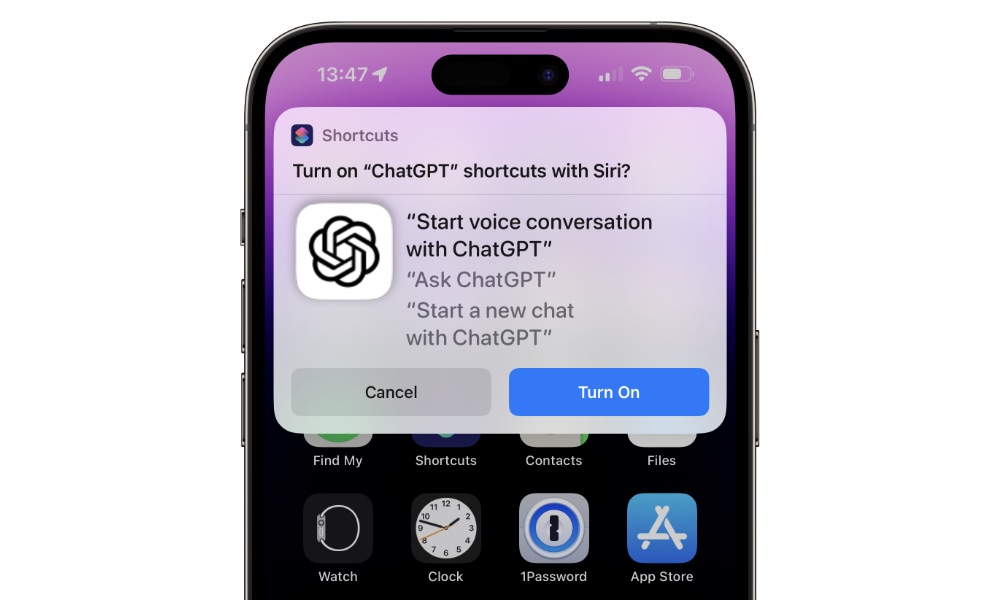The image is a cell phone screenshot, which displays only the upper half of the screen. The top portion of the screenshot has a purple background. Directly below the purple background is a gray square. Inside the upper left-hand corner of this gray square is a smaller black square containing a red and green shape.

To the right of this black square, the word "Shortcuts" appears in gray text. Two lines beneath this, in black text, is a prompt that reads, "Turn on 'ChatGPT' Shortcuts with Siri?" This line is underlined with a very thin, faint gray line.

Below this faint gray line is another square containing a black braid-like circular design. Adjacent to this square, in black text and within quotation marks, it says, "Start voice conversation with ChatGPT." Just below this, there is a gray text in quotation marks that reads, "Ask ChatGPT," followed by another line of gray text in quotation marks stating, "Start a new chat with ChatGPT."

Towards the bottom of this section, there is a gray "Cancel" button situated on the left and a blue "Turn On" button on the right. The rest of the visible portion of the screenshot shows a black background with several app icons at the bottom. The readable app icons include "Find My," "Shortcuts," "Contacts," and "Files." Additionally, there is a row of app icons at the very bottom, including "Watch," "Clock," "1Password," and "App Store."